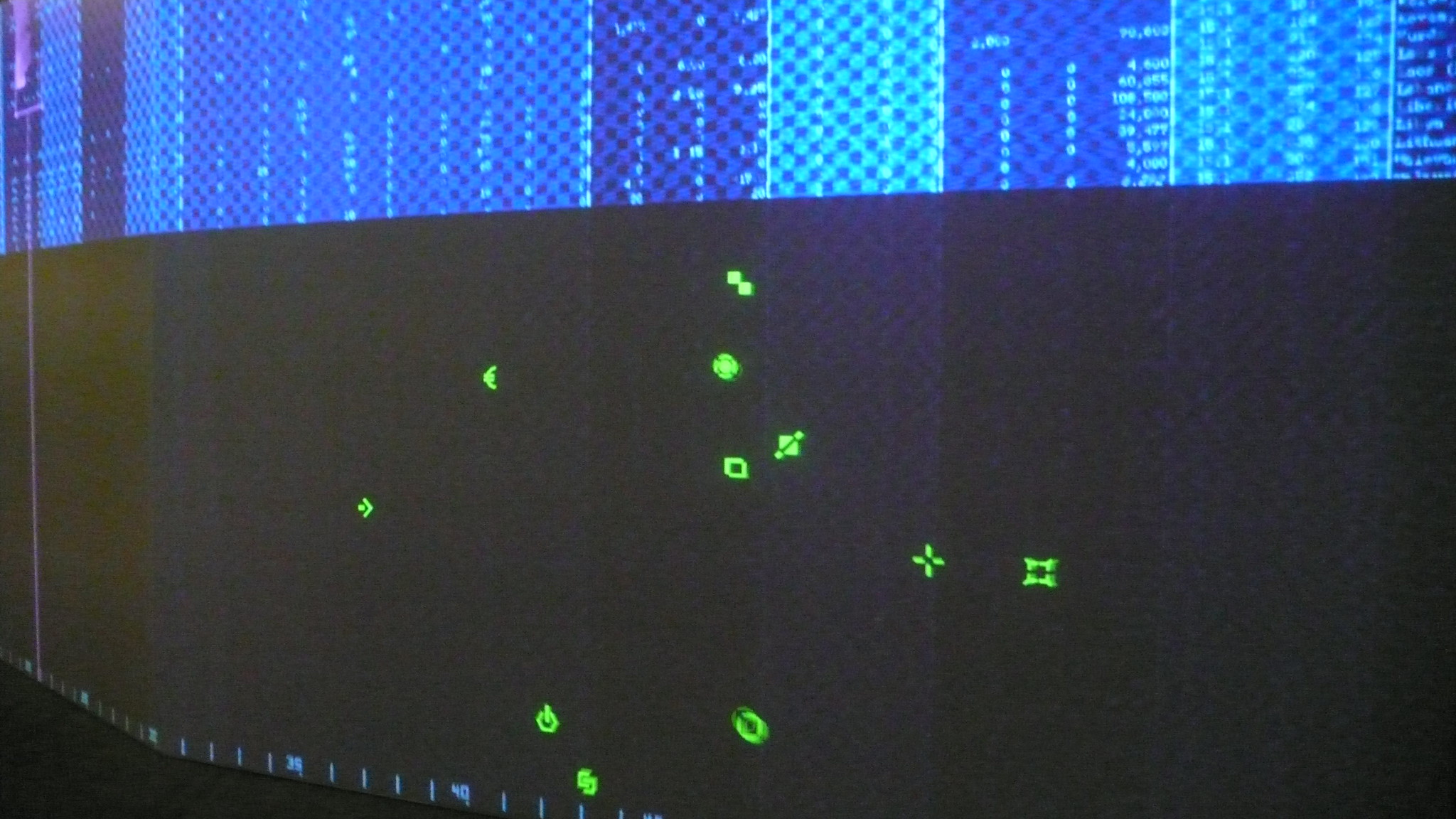The image depicts a large, expansive surface, predominantly showcasing a sleek, suede-like black section at the bottom. Scattered across this black area are various minute, green illuminated symbols, including squares, circles, and arrows. Among these, a distinct power symbol—a circle intersected by a vertical line reaching from the top to its center—is clearly visible. Above the black surface, a row of vibrant blue lights shines through a plastic covering. These blue lights vary in intensity, with some appearing notably brighter than others, creating a striking contrast against the background.